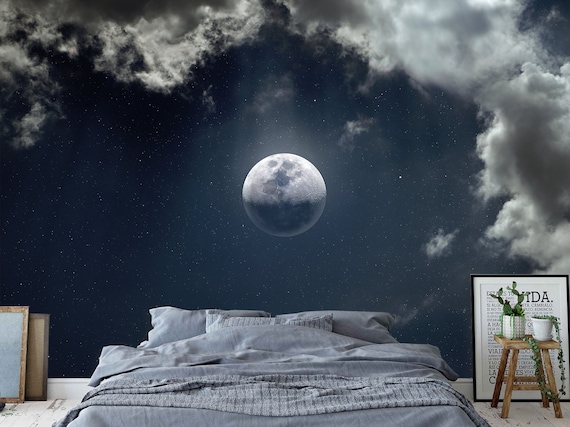In this detailed and stylistic image of a bedroom, the focal point is a large, photorealistic mural on the back wall. The mural, painted in rich, dark blue hues, features a captivating night sky adorned with white dots resembling stars and large, puffy clouds spread predominantly across the top, especially on the right-hand side. At the center of the mural, the moon is depicted in stunning detail, its craters and textures visible, with the top half illuminated to a bright white and the bottom half cast in shadow, as though lit by a hidden Sun.

In the foreground, a bed with light blue blankets, gray bedding, and matching pillows sits low to the floor. The bedding comprises solid gray sheets complemented by a gray and white design on additional layers, adding to the room's cohesive color palette. 

To the right of the bed, a black-framed photograph with white matting and unreadable white text leans against the wall. In front of this frame, a short wooden stool supports two potted plants, adding an element of natural decor to the scene. To the left of the bed, two empty picture frames are also propped against the wall, suggesting a creative or artistic touch possibly from the room's inhabitant. There are no people present in the image, emphasizing the serene and contemplative atmosphere of this meticulously designed space.